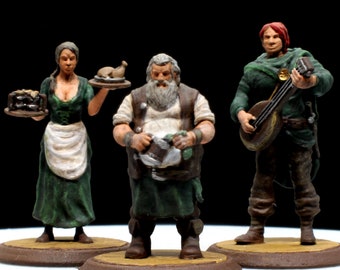This image depicts three intricately painted medieval-themed figurines, each standing on circular brown bases against a white background. On the left is a woman, resembling a Serbian innkeeper, dressed in an ankle-length green gown and a white apron. She has her hair tied back and covered, and she holds two serving trays—one with what appears to be chicken legs and the other with a large pie. In the center is a stout older man, likely a barkeep, with gray hair and a long beard. Adorned in a leather vest, white shirt, green pants, and brown boots, he is intently washing a tankard. On the right is a bard with bright red hair, wearing a green shirt and brown pants, skillfully playing a lute. These figurines appear to be part of a collectible set, capturing a vivid medieval scene.